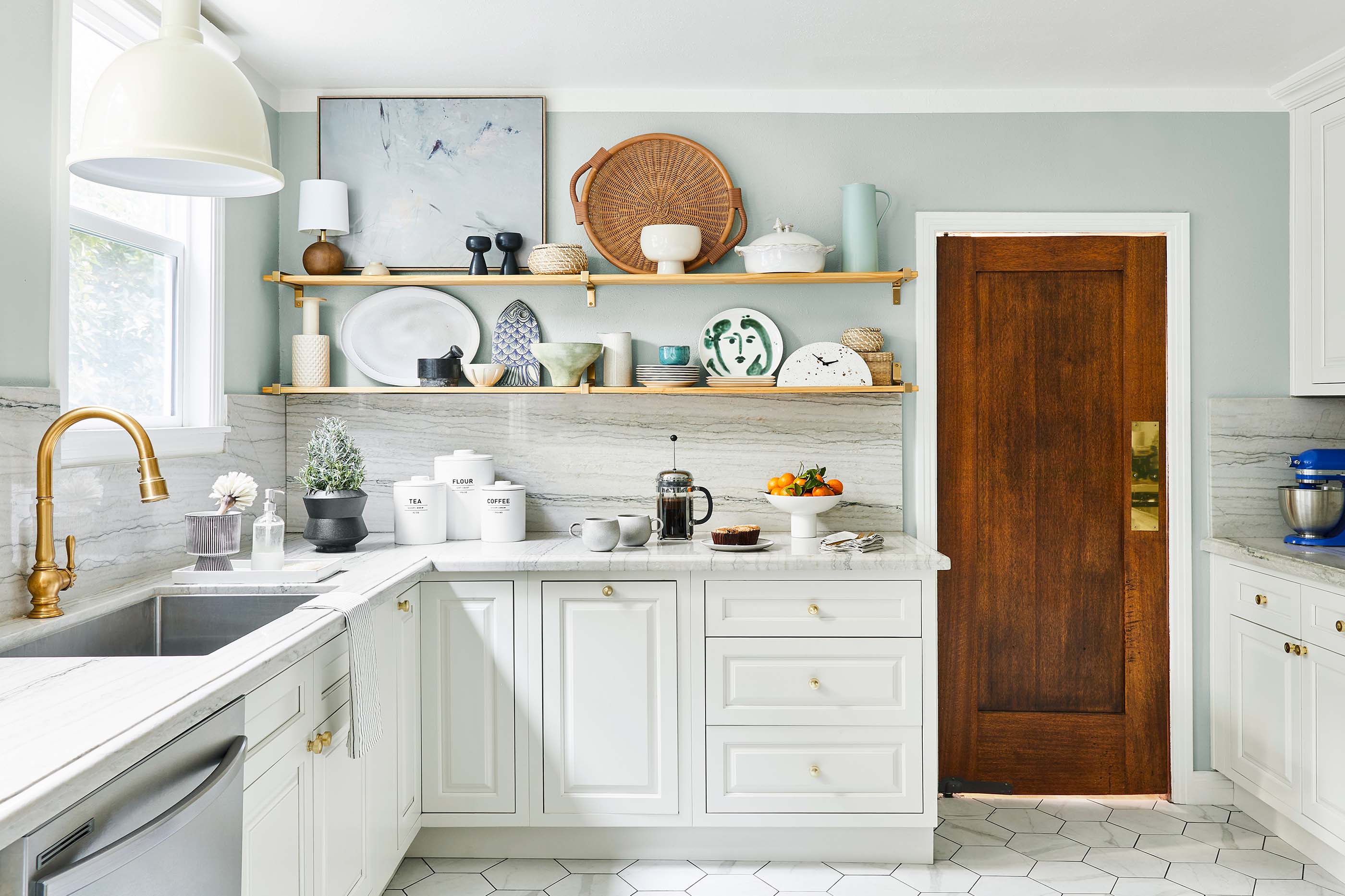This photograph captures an immaculate and stylish kitchen, predominantly adorned in various shades of white, exuding a contemporary and fresh aesthetic. The kitchen features stainless steel appliances, including the top part of a dishwasher visible in the lower left corner. The cabinetry is all white wooden with sleek surfaces, complemented by white marble countertops and a white granite backsplash that together create a cohesive, bright look.

The sink is a large, single-basin recessed rectangle, also made of stainless steel, enhanced by a striking golden copper-colored faucet which adds a touch of elegance. Above the sink hangs a white ceiling lamp, providing ample lighting for the workspace.

Against a very light bluish-gray wall are two light wood-colored shelves arranged horizontally. These shelves are well-decorated with a variety of bowls, plates, and other decorative items, including a mixer and a small tray of fruit, underscoring both beauty and functionality. 

In the background, a rich brown wooden door stands out, accented with a polished brass push plate, adding a subtle contrast and grounding the scene with a hint of traditional charm.